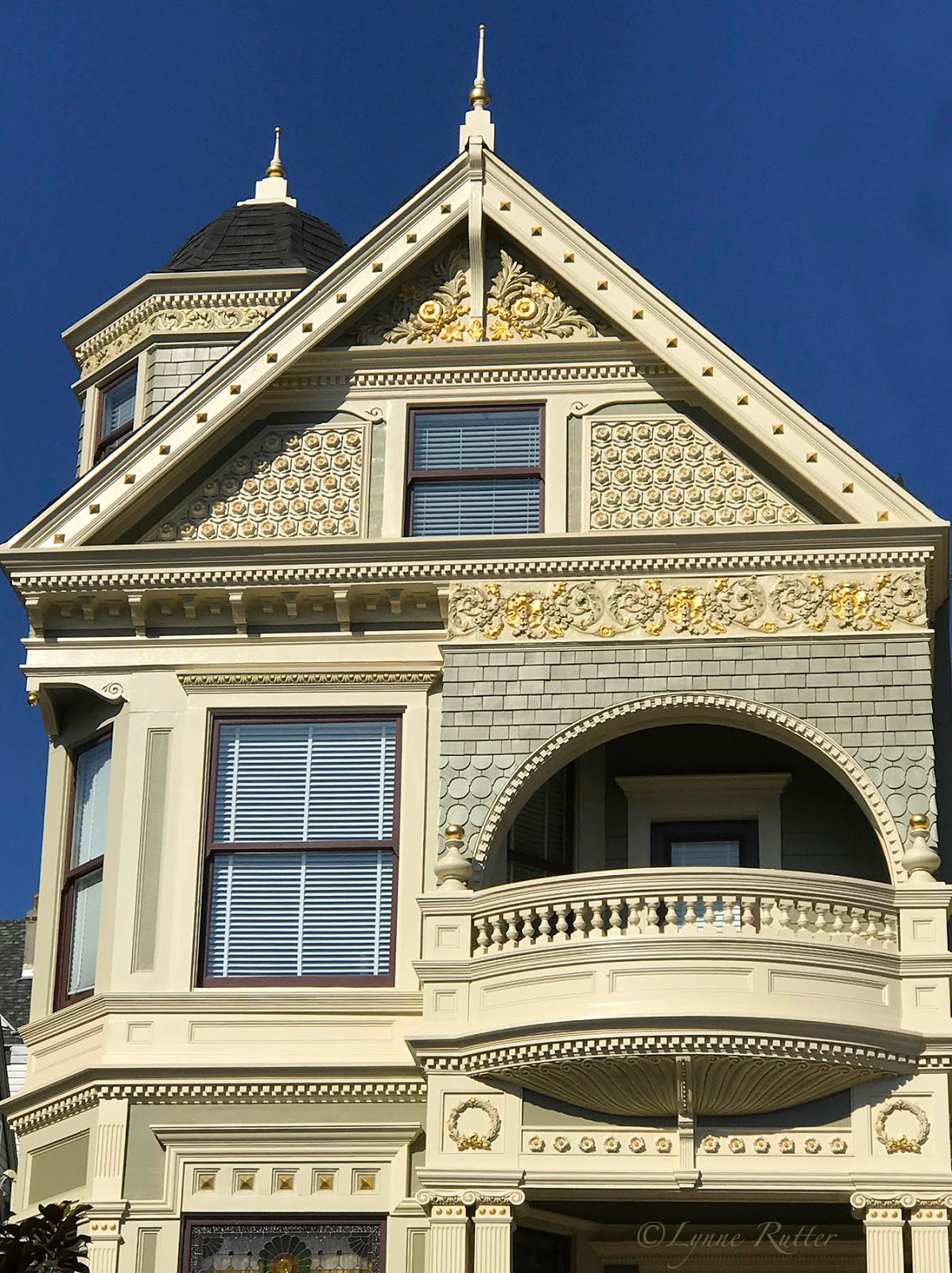This outdoor daytime photograph captures the front facade of a likely century-old, traditional three-story building reminiscent of San Francisco's sophisticated architecture. The building's exterior is primarily light beige or light yellow, with various materials adding texture and detail. A notable feature is the rounded archway above the second-floor balcony, which is adorned with gray or silver bricks and intricate curved flower decorations with gold accents. The balcony itself is constructed from similar gray tiles. The lower left corner of the image contains a copyright mark for Lynn Rutter.

On the right side of the building, there’s an arched opening with columns leading to the balcony, while the left side features a double-paned window with white drawn shades. Another window's side profile is visible as the house rounds toward the left. The top of the structure shows a triangular-shaped attic with a single window surrounded by filigree, beehive patterns, and emblematic details. Dominating the left side of the building is a domed rooftop, black in color with white tips. All of this is set against a striking royal blue sky, capturing the building's grandeur and intricate designs under the bright, sunny day.